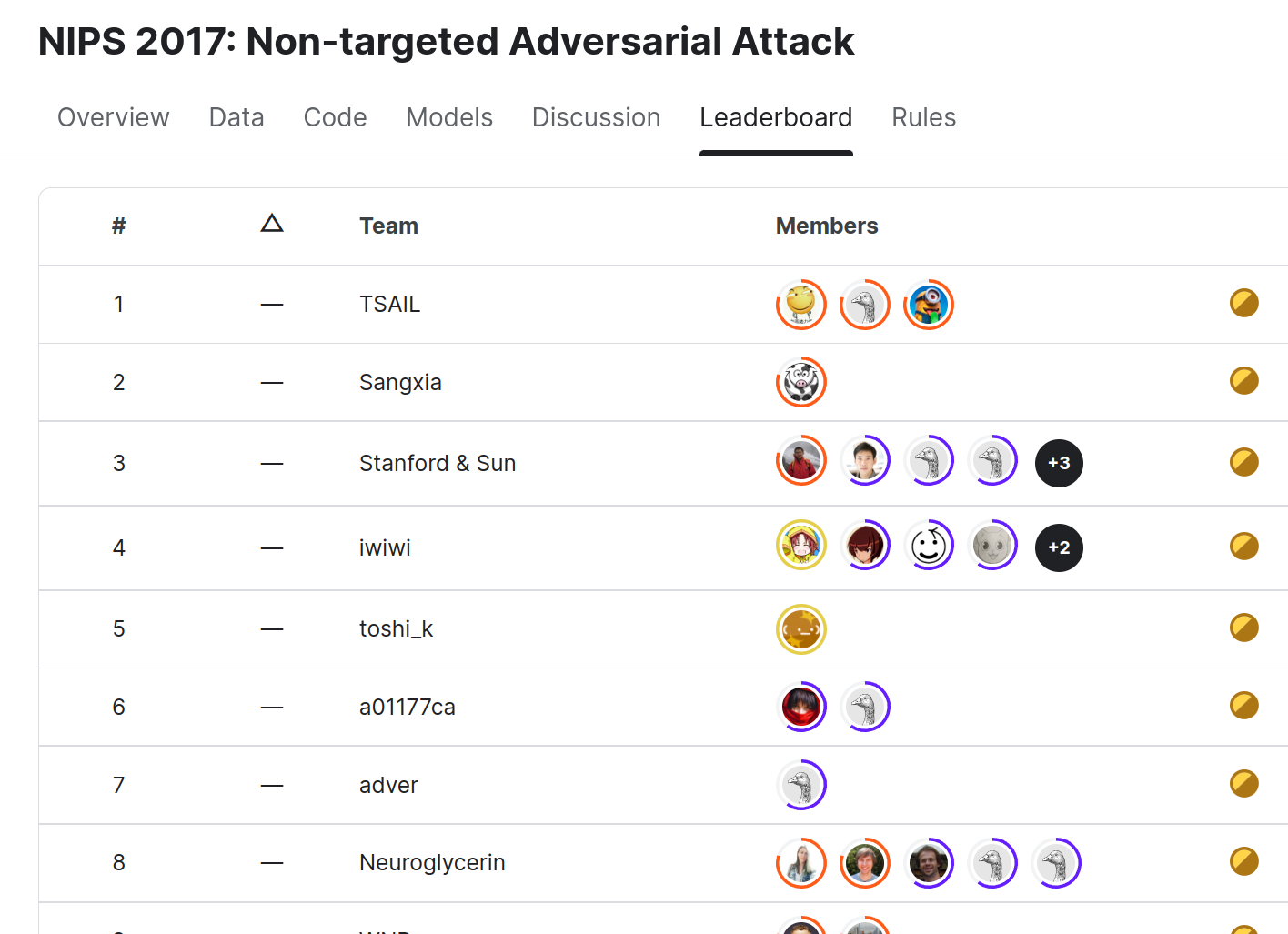The screenshot displays a leaderboard for a game or competition, specifically titled "NIPS 2017 Non-Targeted Adversarial Attack." The top-left corner of the image features this title prominently. Below the title, there is a navigation bar with several tabs labeled "Overview," "Data," "Code," "Models," "Discussion," "Leaderboard," and "Rules." The "Leaderboard" tab is highlighted with an underlined, black line, indicating the current view. The leaderboard itself is arrayed on the left side, featuring rankings numbered one through eight. Each rank lists various team names along with member profiles, which are represented by either profile pictures or gaming avatars.